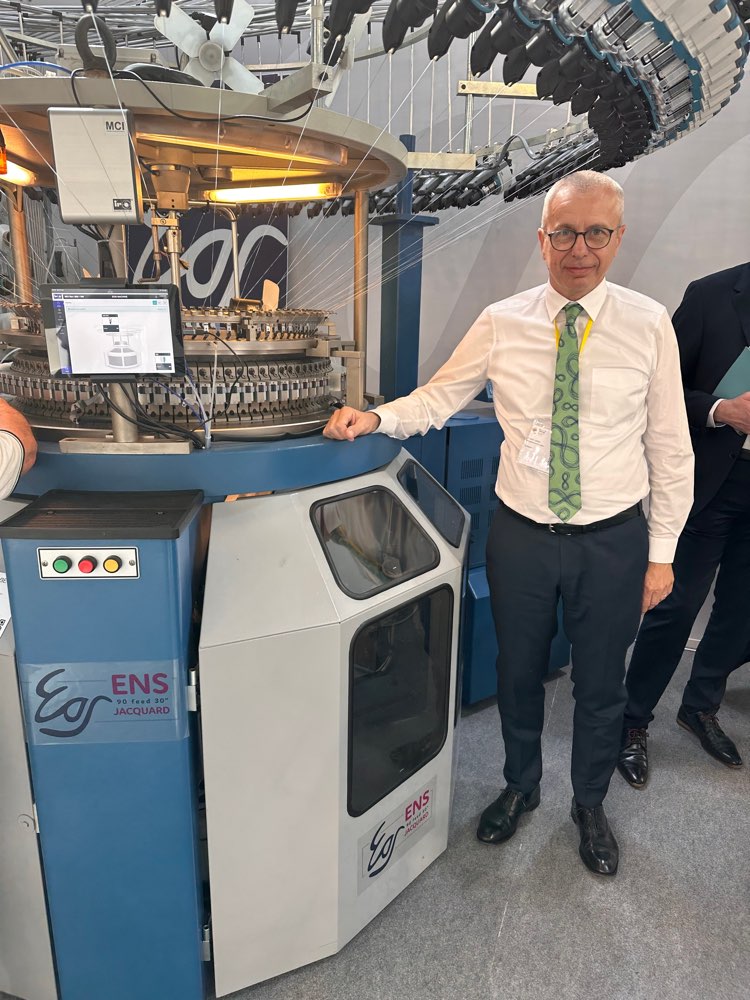In an indoor setting, a distinguished man in his 50s, wearing a cream-colored dress shirt, a green tie, black pants, black shoes, and eyeglasses, stands prominently next to a large, complex industrial machine. The man is gazing directly at the camera with one arm propped on the machine, exuding confidence and poise. The machine, primarily gray and blue, features a central circular portion housed within a glass enclosure and is labeled with "EOS" and "ENS" in capital letters. A sign on the machine also includes the text “90 feet, 30 inches, Jacquard.” The machine has three colored buttons on the side: red, green, and yellow. The scene includes additional people in the background, partially visible, one holding a green book. The setting and the advanced-looking machine evoke a sense of high-tech industry, possibly related to manufacturing or scientific research.